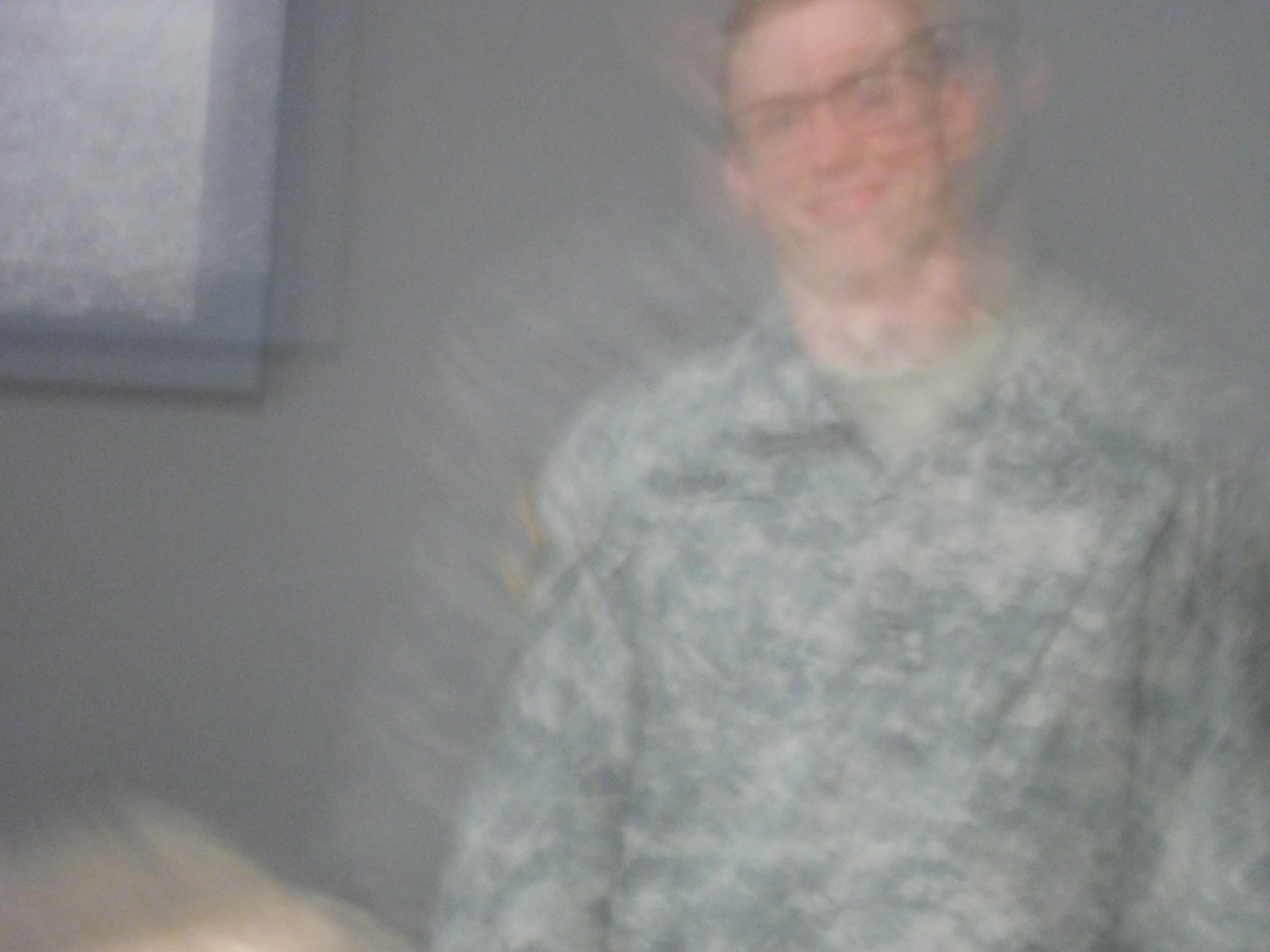The photograph is a blurry image of a Caucasian man with very short hair, smiling and facing the camera. He is wearing glasses with a frame on the top part but not on the bottom lens. The man is dressed in a beige and green camouflage military uniform, known as BDUs (Battle Dress Uniforms), with a light green T-shirt underneath. The uniform includes a camel-colored jacket with a badge on the right arm, though the details are difficult to discern due to the blurriness. The photo seems to have been taken indoors, with the left side of the image featuring the edge of a window or mirror frame, likely gray in color. Below this, in the bottom left corner, there's an indistinct beige or orange-yellow object. A bed and possibly a small window can be seen in the background, illuminated by light filtering through. The image appears to suffer from camera shake, causing the man to appear double or even triple exposed.